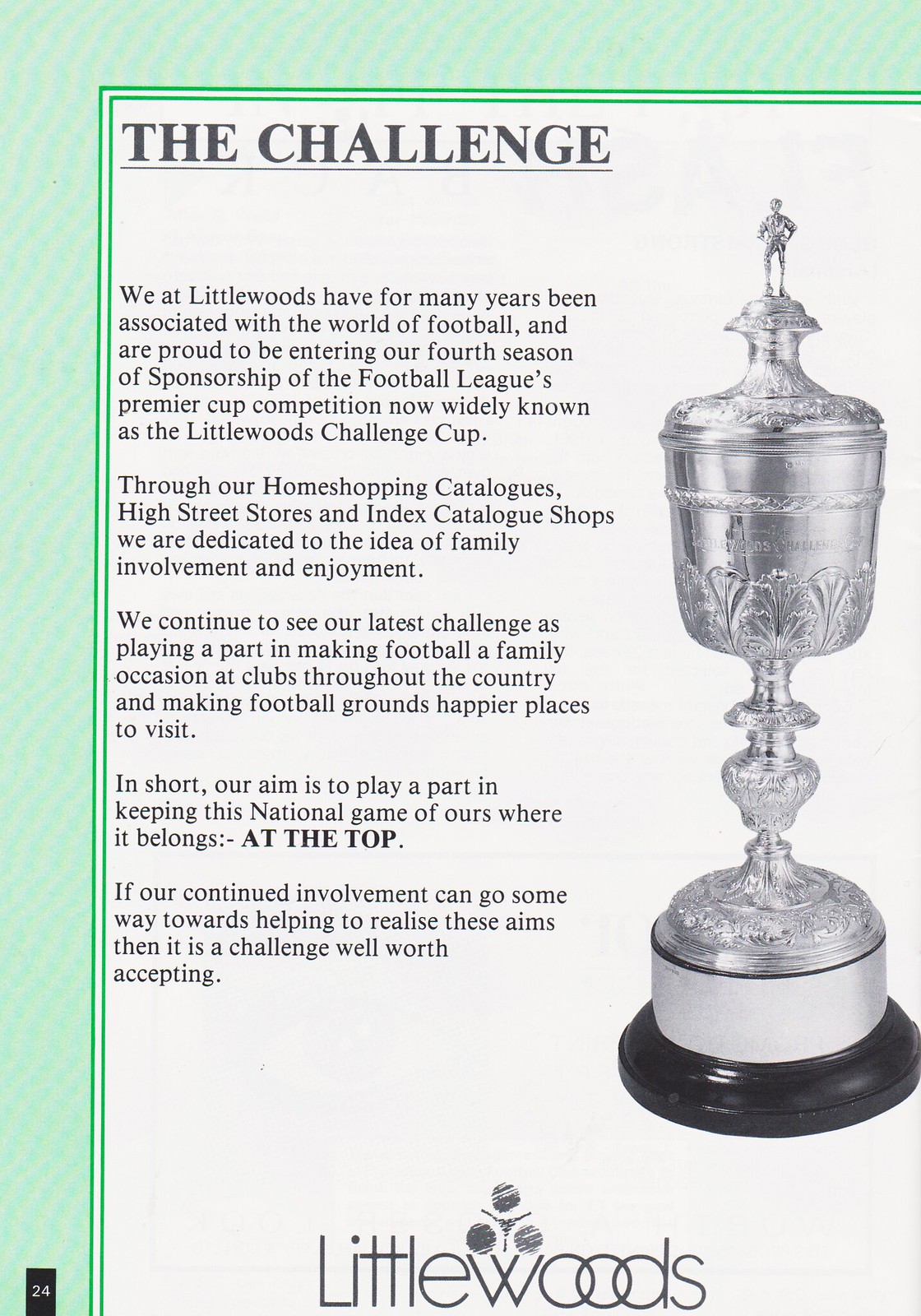The image features a page from a magazine or program, designed in portrait orientation. The layout includes a white text box bordered by green stripes—light green on the outside with a darker green rule on the inside—along the top and left sides. The main content, titled "The Challenge," is printed in black text against a white background. 

To the right of the text box, occupying approximately two-thirds of the vertical space, is a photograph of a tall silver trophy with a soccer player on top and a black base at the bottom. Below the trophy image, the text reads "Little Woods" alongside the company's logo, which includes three circles above a pyramid shape in a lightweight black font.

The text discusses Little Woods' longstanding involvement in football, entering their fourth season sponsoring the Football League's Premier Cup competition, now commonly referred to as the Little Woods Challenge Cup. It elaborates on their commitment to making football a family-friendly event through their home shopping catalogs, high street stores, and index catalog shops, aiming to enhance the football experience and maintain the national sport's prominence. At the bottom left corner of the page, within the green border, a black rectangle with white text indicates the page number: 24. 

Overall, the page effectively combines detailed textual content and visual elements to convey Little Woods' mission and sponsorship in a classic print publication style.